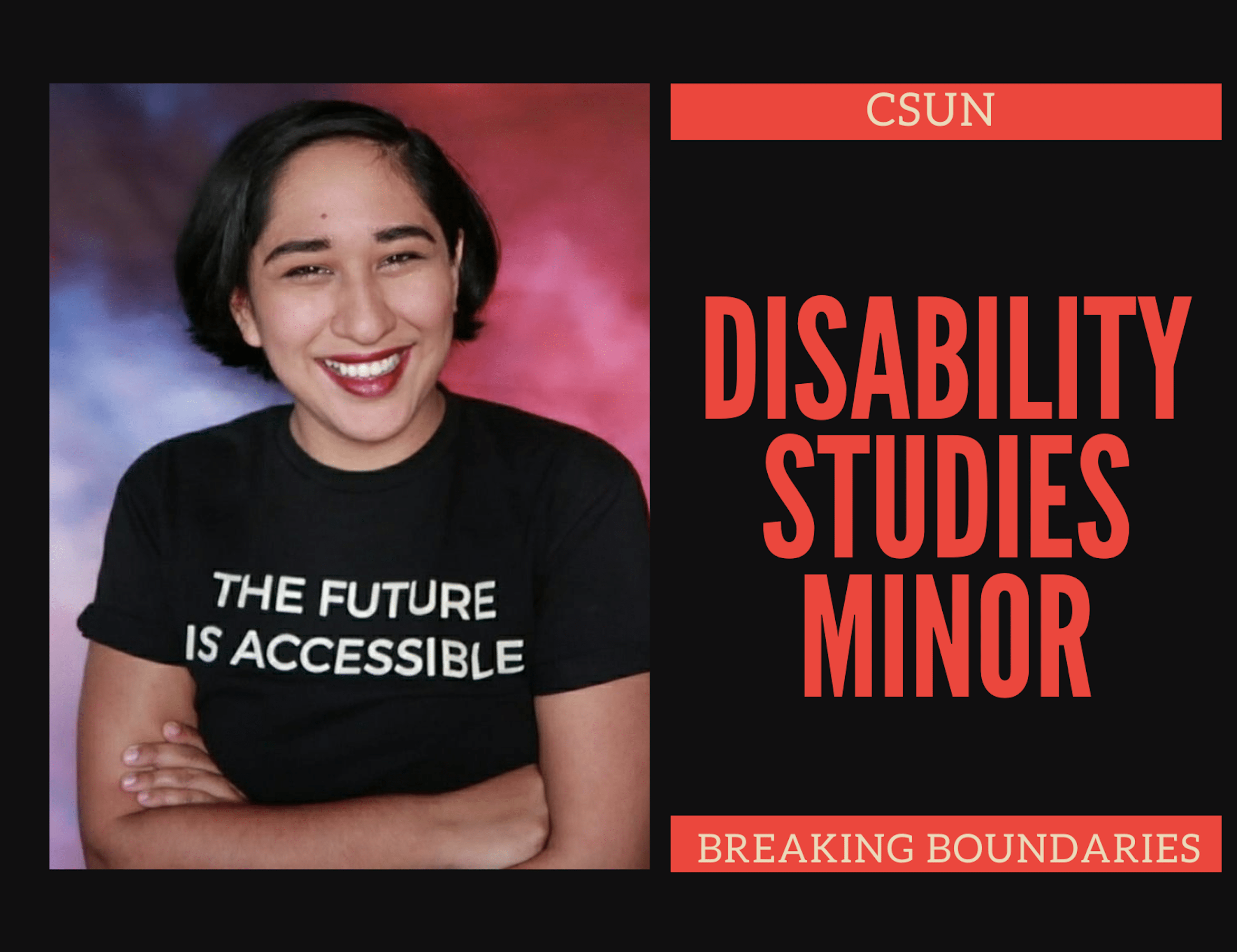The image features a black background and is divided into two sections. On the left side, there is a photograph of a woman with short, ear-length black hair. She has thick eyebrows, prominent cheeks, a pronounced chin, and is smiling broadly, showing her top teeth. She wears red lipstick and is dressed in a black t-shirt with the text "THE FUTURE IS ACCESSIBLE" written in all caps white letters. Her arms are crossed over her chest, and she is visible from the waist up. The background of her photo is a dynamic blend of red and blue, resembling a tie-dye pattern.

On the right side of the image, there is text on a black background, divided by two red bars. At the top, a red bar contains the acronym "CSUN" in white letters. Below this bar, the words "DISABILITY STUDIES MINOR" appear in large, all-caps red text, each word on its own line. At the bottom of the image, another red bar holds the phrase "BREAKING BOUNDARIES" in white, all-caps text.